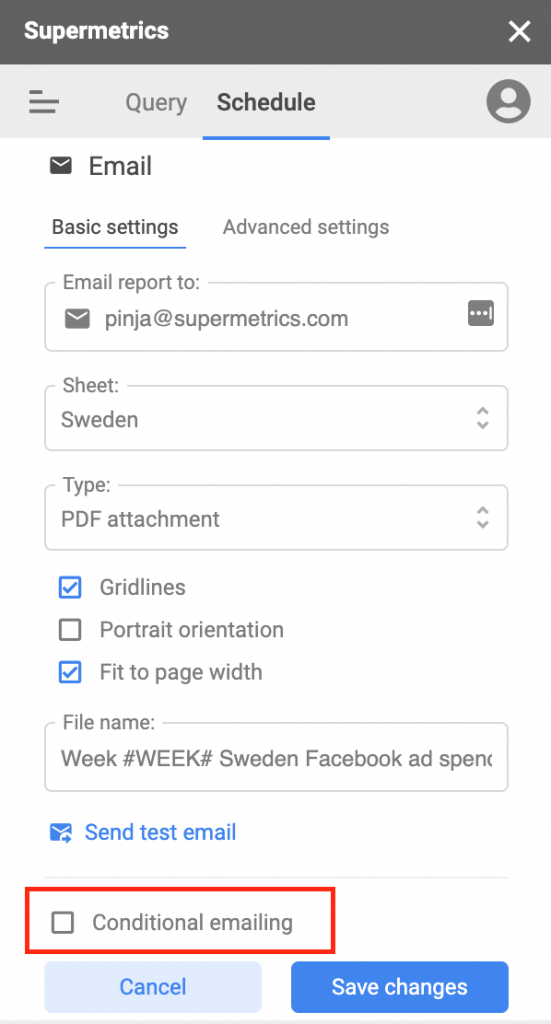**Detailed Image Caption:**

The screenshot appears to be from a smartphone displaying an interface of the Supermetrics app. The top section is a gray bar with the word "Supermetrics" in white lettering, with a capital "S." On the far right of this bar, there is a white "X". 

Below this, there is a light gray quadrant with three horizontal gray bars on the left-hand side— a small one, a longer one, and a slightly shorter one. To the right of these bars, the word "Query" is written in capital letters (Q-U-E-R-Y). Next to it, the word "Schedule" appears in white with a blue underline. Adjacent to this is a small round gray circle, which appears to be an icon of a person.

Beneath this section, on the left, is a gray envelope icon next to the word "Email" with a capital "E". Below is another label, "Basic Settings" with a capital "B," separated by a blue line. Next to this, in light gray, is "Advanced Settings" with a capital "A," also separated by a blue line.

Further down, the text "Email Report to:" is shown in gray. A gray border surrounds this text and stretches horizontally, creating a box-like structure. Within this box, the email address "pincha@supermetrics.com" appears in gray lettering. To the right, there's a gray box with three white vertical dots and a vertical white line.

Another gray box sits below, outlined with a word "Sheet:" in gray. Inside this box, "Sweden" is written in gray. To the right, a vertical gray arrow points up and down.

Below this, there is a section labeled "Type:" followed by "PDF" and the word "attachment," accompanied by another up and down gray arrow.

The next section features three small boxes. The first box is blue with a white checkmark, and next to it is the word "Gridlines" in gray. Below, a gray-bordered box with white inside is labeled "Portrait Orientation" in gray next to it. Below this, another blue box with a checkmark next to "Fit to Page Width" in gray.

Another boxed section below contains the word "File Name:" in the left-hand corner. Inside this section, in dark gray letters, are "WEEK#WEEK#Sweden Facebook Ads", with the last part cut off.

Near the bottom, there is a blue box with a white plus icon beside the words "Send Test Email" in gray. Below this, a red-bordered box with "Conditional E-Mailing" written next to it in gray.

At the very bottom, there are two rectangular buttons with curved edges. The left button is light gray with "Cancel" in dark blue. The right button is dark blue with "Save Changes" written inside, both with a gray underline at the bottom.